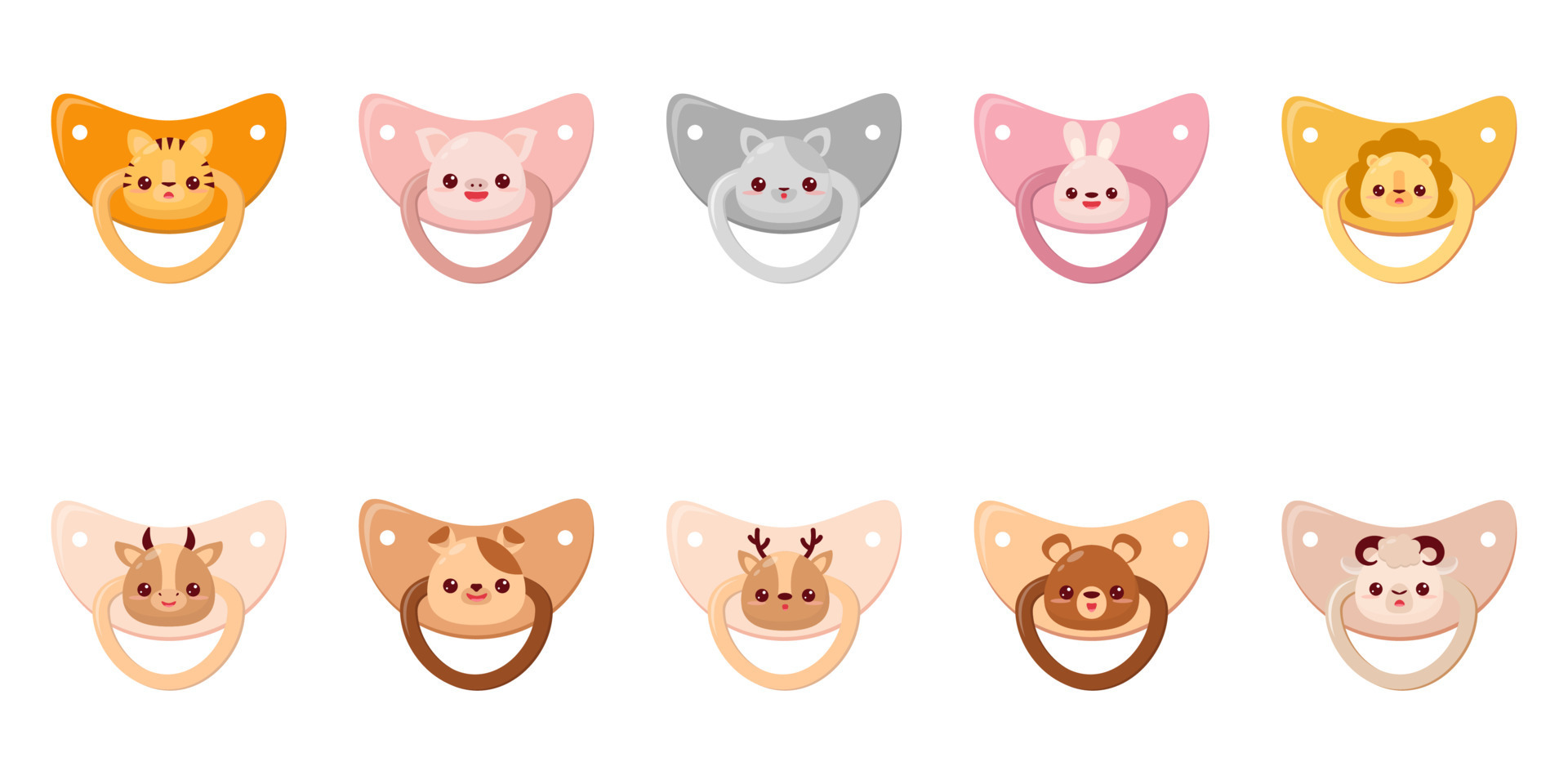The image features ten cartoon-style pacifiers, commonly referred to as binkies, arranged in two uniform rows of five against a white background. Each pacifier is adorned with a cute, child-friendly animal illustration at its center, including rabbits, reindeer, pigs, kittens, lions, bears, goats, sheep, and dogs. The color palette is varied and inviting, showcasing hues of orange, pink, blue, yellow, brown, and beige. The pacifiers are displayed with their handles facing downward, and the overall arrangement and design suggest a catalog entry or display intended for baby product selection.